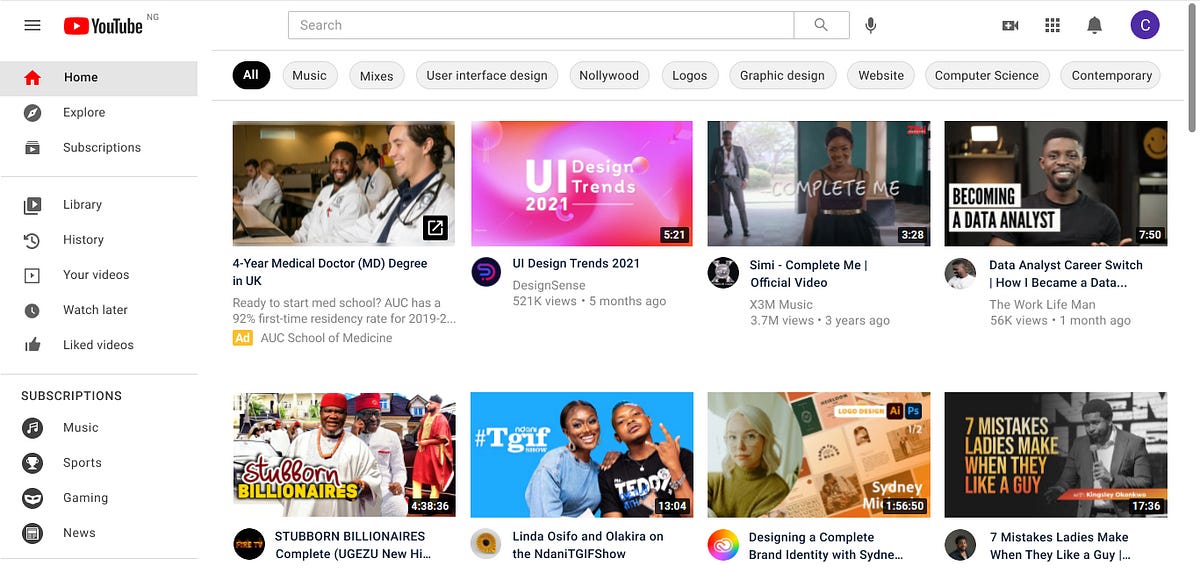This is a detailed screenshot of a website's home page, primarily YouTube, featuring a clean design on a white background. At the very top, a thin light gray horizontal line stretches across the frame, adding subtle separation.

On the left side, just beneath this line, is a dark gray hamburger menu. Adjacent to the menu, the recognizable YouTube logo is prominently displayed: a red rectangle with rounded corners and a white right-pointing triangle inside. To the right of this logo, the black text "YouTube" is clearly visible, followed by light gray uppercase text "NG" positioned slightly above and to the right.

Moving rightwards into the larger negative space, there is a white search bar outlined in light gray. Inside the search bar, the placeholder text "search" is in light gray on the left, followed by a light gray vertical separator line. To the right of this separator, a light gray magnifying glass icon is visible, indicating the search function. Outside the search bar, next to it on the right, a dark gray microphone icon suggests voice search capability.

Further to the right after more negative space, a series of functional icons follows, starting with a dark gray cinema camera icon with a white plus sign inside, indicating the option to upload a video. Next, there's a 3x3 grid of dark gray squares, likely indicating a menu or additional options. Following this, a dark gray bell icon for notifications is displayed. The section concludes with a user avatar, represented by a purple circle with an uppercase white "C" inside.

Beneath this main navigation area, another thin light gray horizontal line separates it from a row of category badges. The first badge is a black pill-shaped button with white "ALL" text. The subsequent badges, all pill-shaped with dark gray text and thin dark gray outlines, include categories labeled "Music," "Mixes," "User Interface Design," "Nollywood," "Logos," "Graphic Design," "Website," "Computer Science," and "Contemporary."

These elements collectively contribute to a clear and user-friendly interface design on the home page.